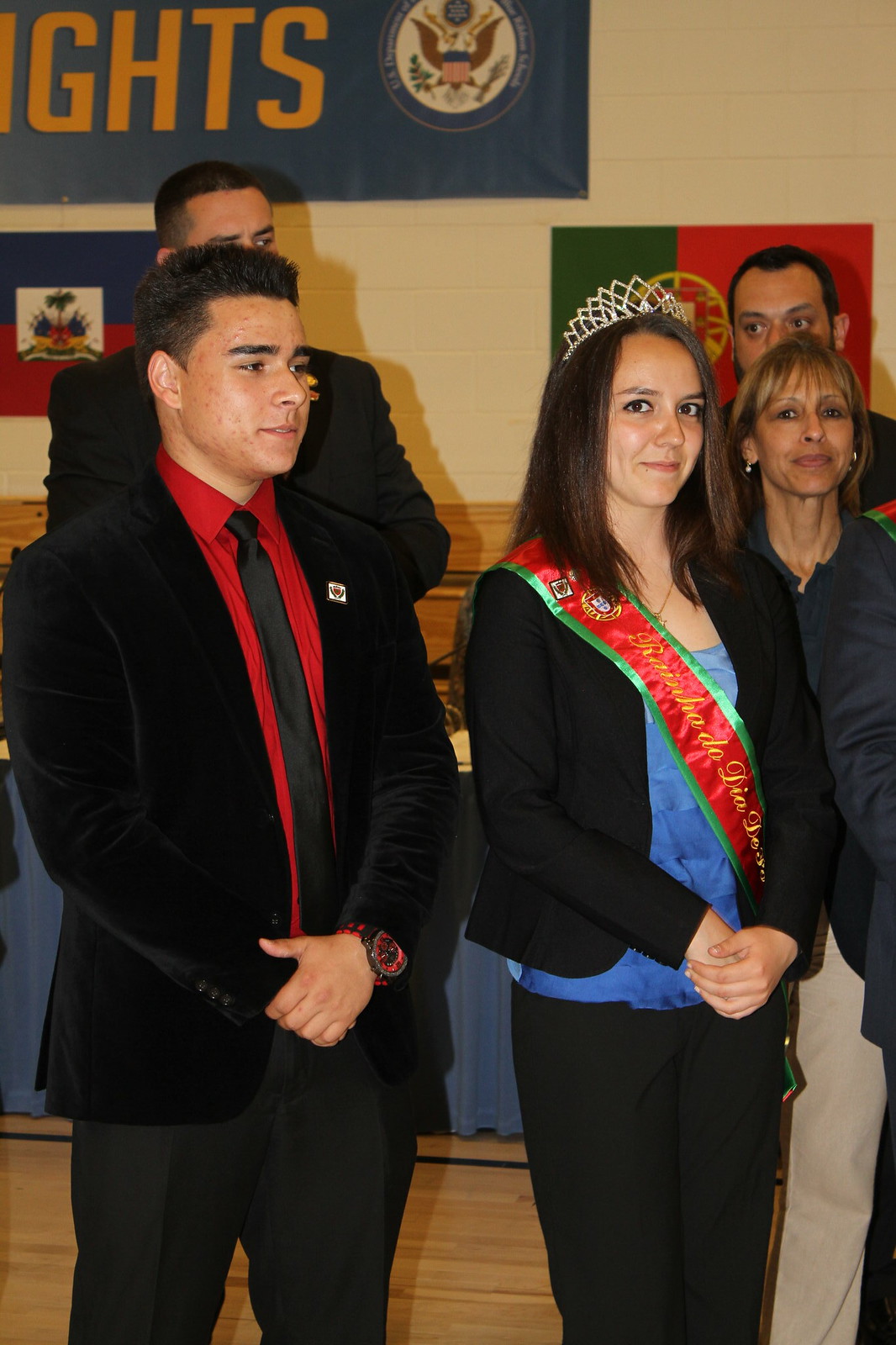In a well-lit community center or school gymnasium, this image captures a formal ceremony or presentation with a white back wall adorned with a large blue banner featuring the American seal and the letters "G.H.T.S." in yellow text. Alongside the banner are additional flags, including one that is blue and red, and another that is green and red with a yellow circle. In the foreground, the focus is on a man and a woman dressed in formal attire. 

The man on the left is wearing a black suit with a red dress shirt, a black tie, and a red and black watch on his left wrist. He has short, neatly styled black hair and a small pin on his lapel. Beside him stands a woman with short brown hair, a black blazer over a blue blouse, and a red and green sash with yellow text. She is adorned with a tiara, and both individuals have their hands clasped together. In the mid-background, five people, including three predominantly visible individuals, are positioned in support. The setting and the attire of the subjects suggest a celebratory or significant community event.